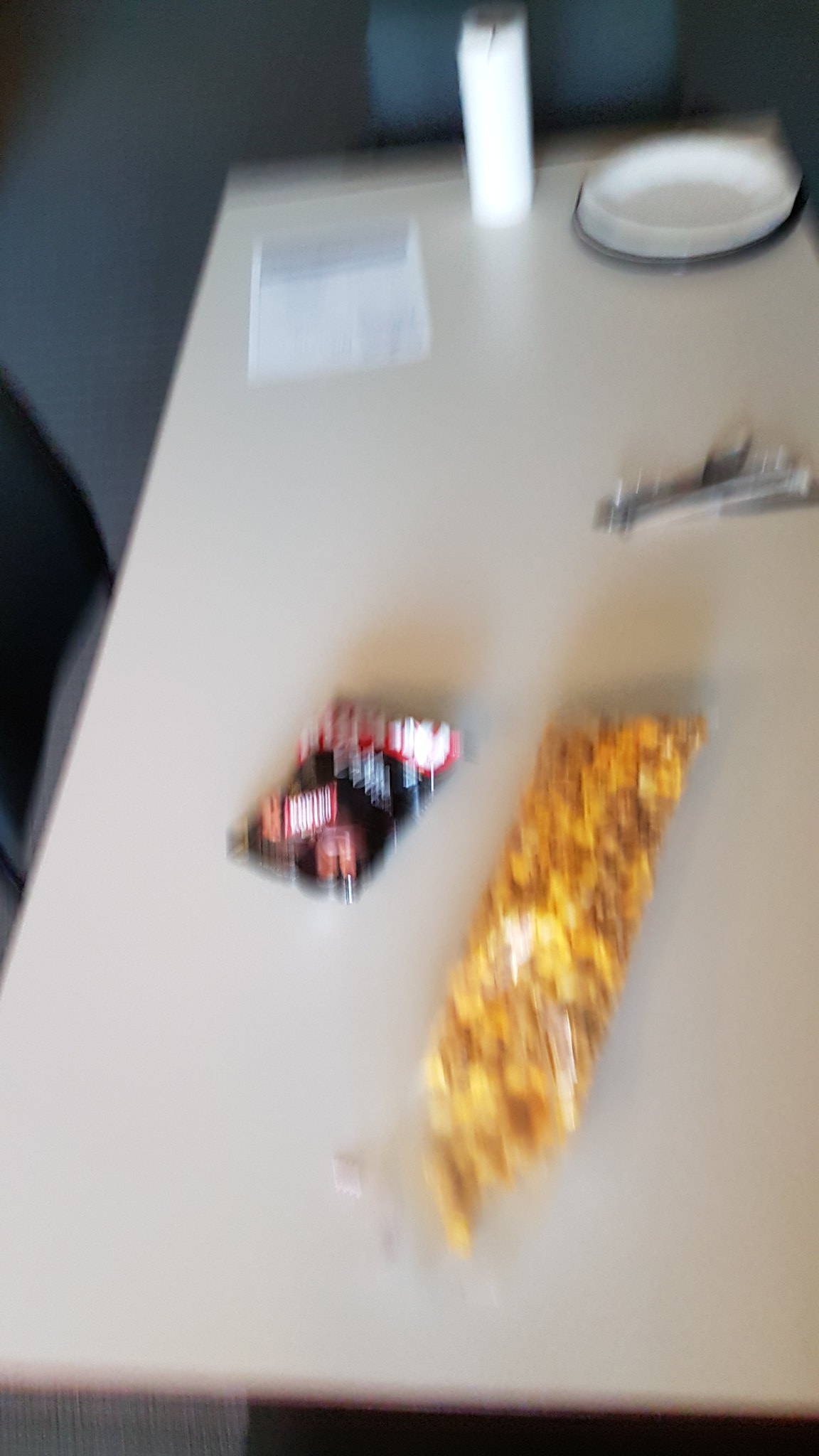This image, captured in portrait orientation, portrays a slightly skewed and out-of-focus scene, possibly due to camera movement or low lighting. The primary focus is a white rectangular table viewed from above. In the foreground, there's an open, clear cellophane bag filled with yellow and brown popcorn, potentially caramel corn. To the left of this bag lies another package, black and silver, with unreadable red and white writing. 

Towards the middle of the table, we see indistinct silverware, likely including a spoon among other utensils. Further up, positioned to the right, is a stack of plates: the top one is entirely white, while the one beneath it is white with blue detailing. On the left side of the table lays a white piece of paper, adorned with darker writing in various sections – at the top, middle, and bottom right corner, though the text is illegible. 

In the background to the right, there's a portion of a chair with a black backrest, and next to it, there's a vertical gray pole extending upward.